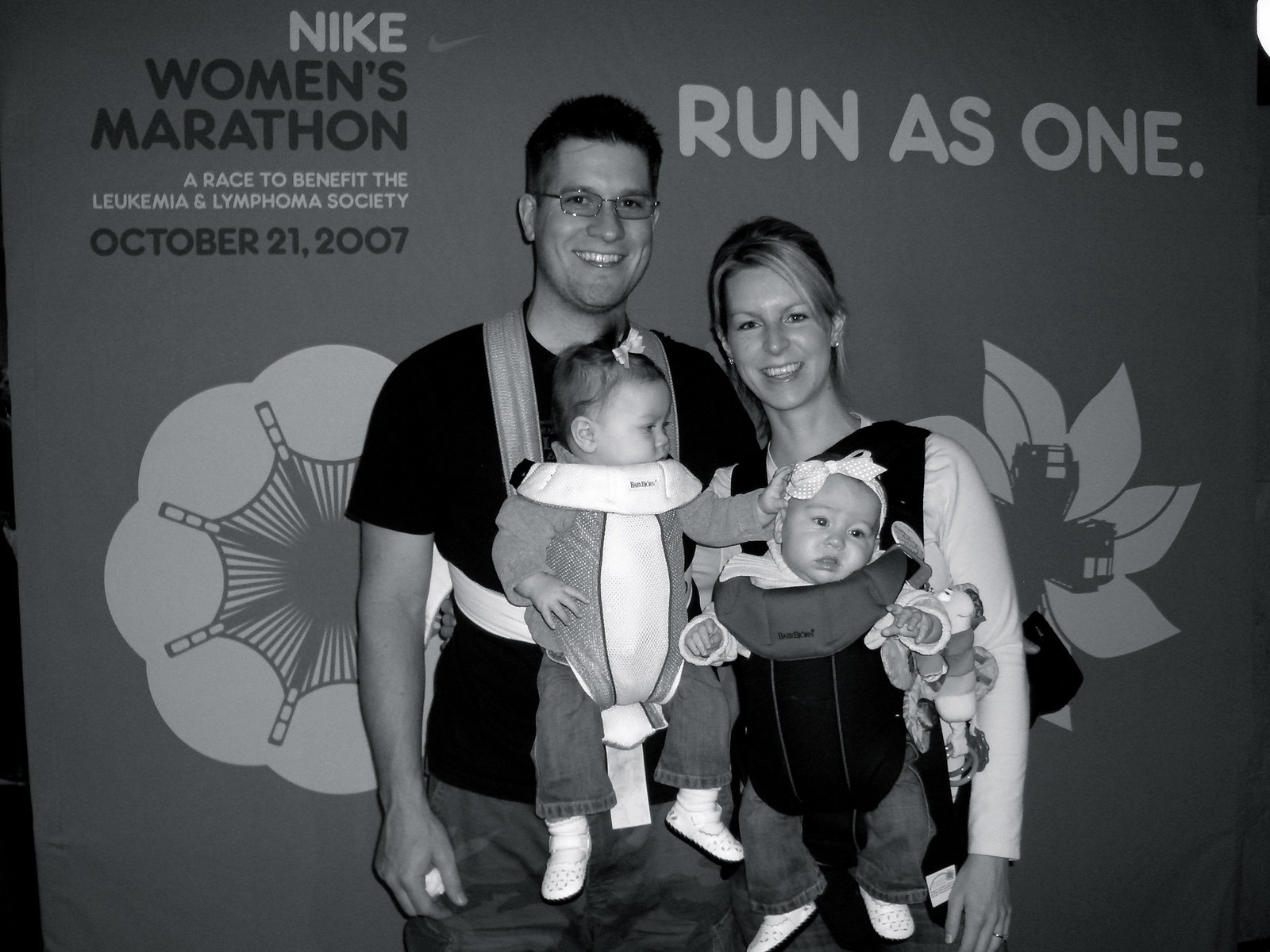In this black-and-white landscape-oriented poster for an upcoming event, a smiling young couple stands at the center, each carrying a child in a front-facing baby carrier. The man on the left has dark hair, wire-rimmed glasses, and wears a dark t-shirt and pants. The woman on the right, in her 20s, has blonde bangs with her hair pulled back and is dressed in a dark black vest over a white long-sleeved shirt. Both children, one appearing to be a boy and the other a girl, each wear a white bow on their heads. The little girl, in a dark top, touches the boy's head, while both babies gaze at the camera. In the backdrop, a gray mural filled with floral emblems sets the scene. Prominent white text on the top right reads "Run as One," while the top left features "Nike Women's Marathon" in black letters, followed by "A Race to Benefit the Leukemia and Lymphoma Society" in smaller white text, and the event date, "October 21, 2007," in slightly larger text. The photographic style of representational realism captures the hopeful spirit and solidarity of the event.